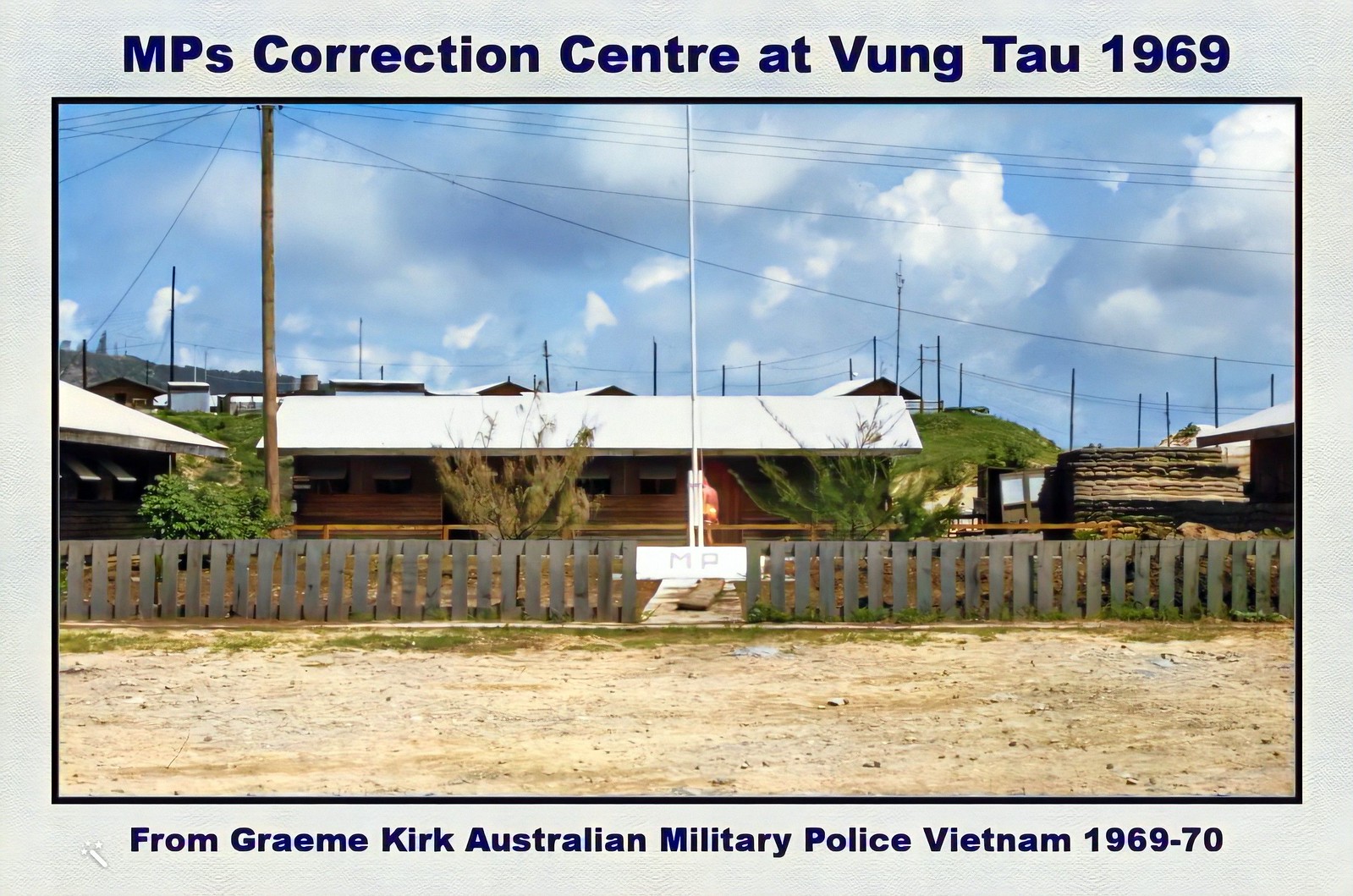This is a wide rectangular image framed with a digitally textured white border. At the top, the caption reads in bold dark blue letters, "MP's Correction Center at Vung Tau 1969," while the bottom caption reads, "From Graham Kirk, Australian Military Police, Vietnam, 1969-70." The central photo is bordered by a thick black frame and depicts a sandy light brown surface with patches of green grass. A waist-high wooden fence with a central entrance supports a white board reading "MP." In the background, a wide wooden brown building with a white triangular roof is visible, flanked by large trees, a prominent bush, multiple telephone poles, and various cables. In front of the building is a bunker-like structure made of rocks, along with other smaller buildings and wood piles. The scene is set under a blue sky with white puffy clouds.